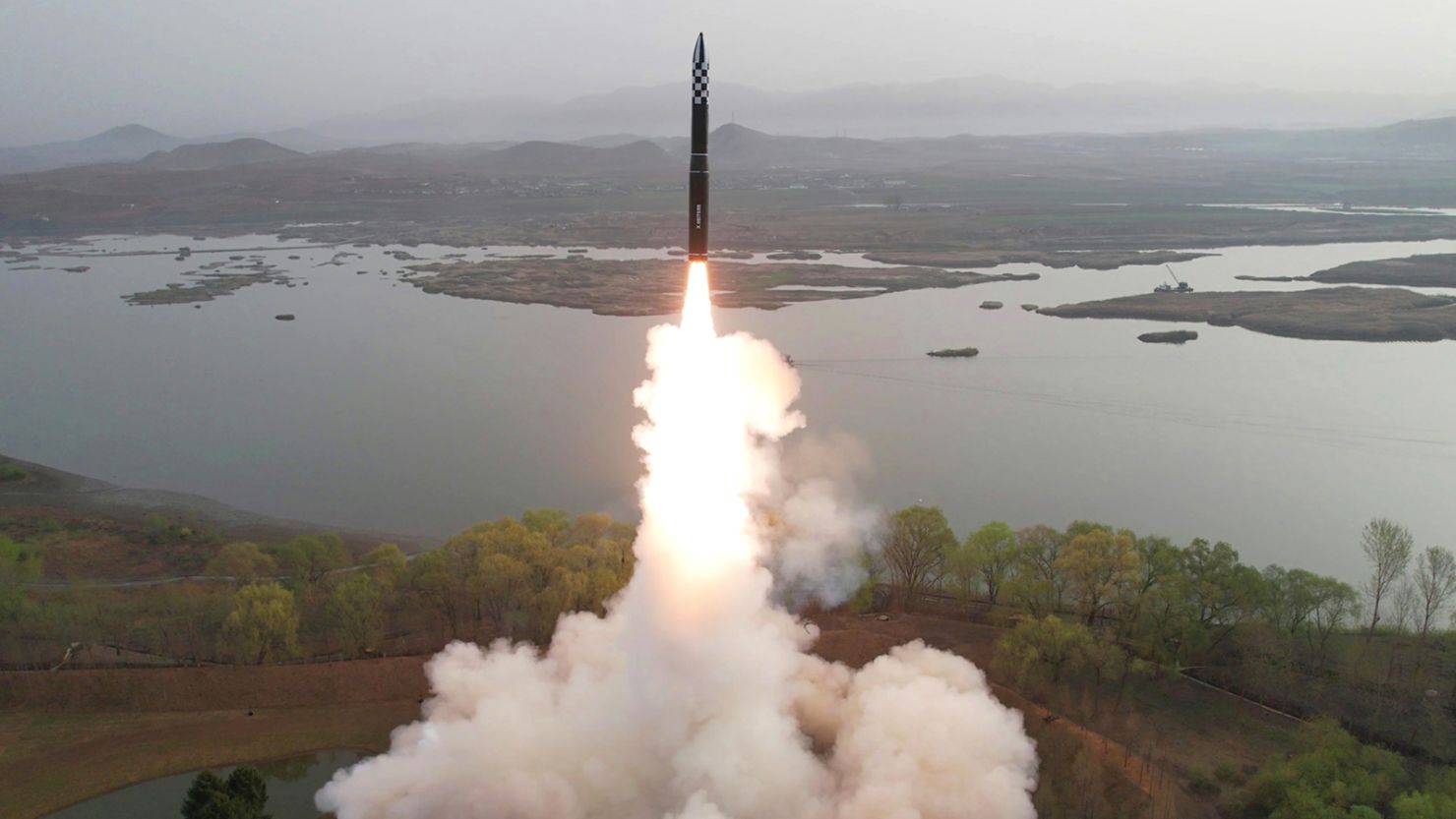The image captures a small rocket launching into the sky, featuring a distinctive black and white checkerboard pattern near its top. The rocket's base emits a fiery plume, propelling it upwards amidst a large cloud of smoke. The rocket resembles a missile, lacking apparent passenger windows, and bears an indeterminate white text on its side, visible yet unreadable from the current perspective.

The surrounding landscape appears desolate, characterized by expanses of water and several scattered islands. In the background, hills are faintly visible. A boat or some sort of vehicle can be seen on the water, and far into the distance, there might be structures such as houses. Trees with yellowing leaves, suggesting an autumnal scene, dot the area around the launch site, which has a generally brownish, non-lush terrain. The overall atmosphere is misty and foggy, imparting a gray, desolate vibe to the scene.